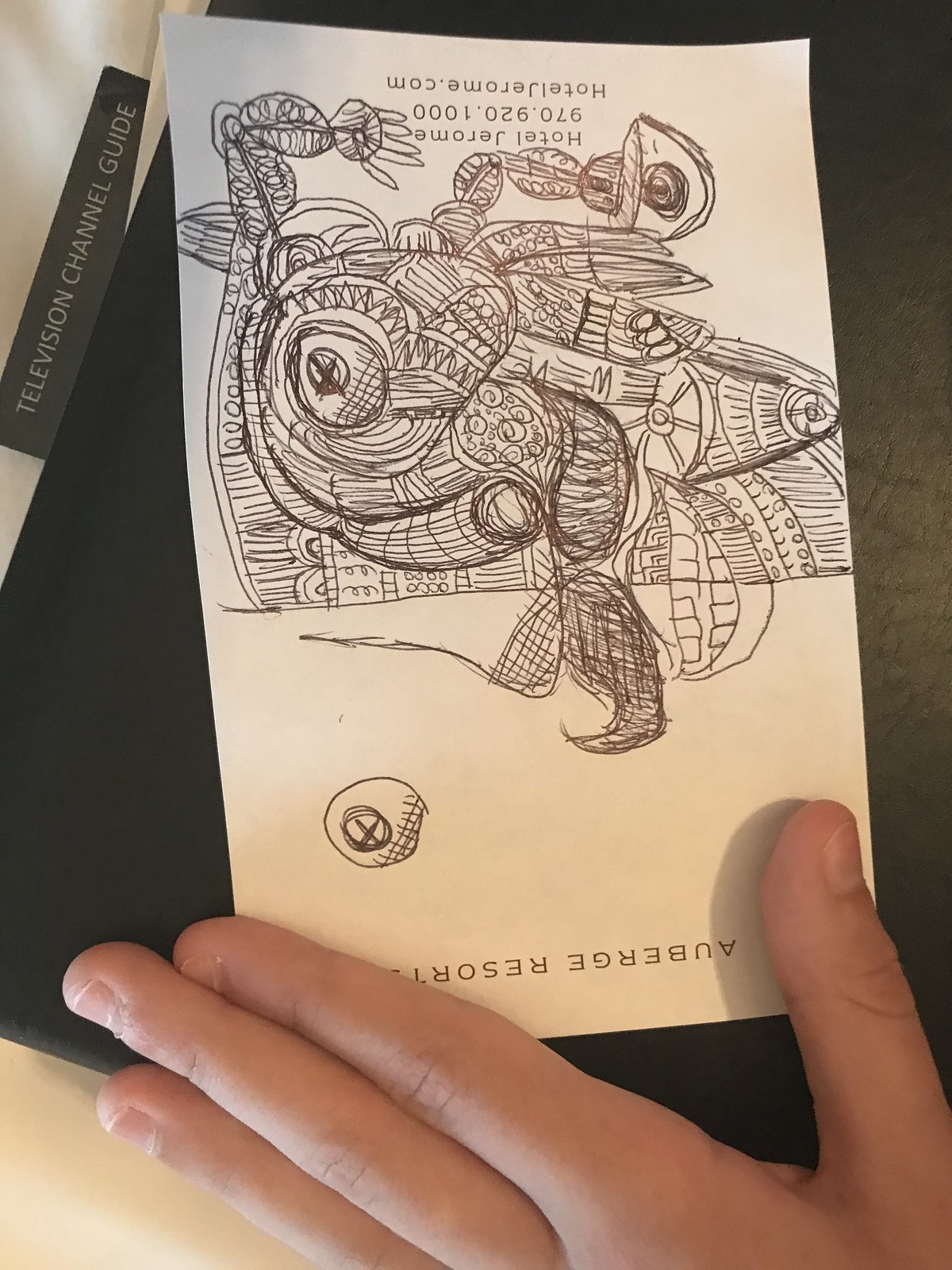A detailed photograph captures an intricate doodle on a piece of paper, presumably made by a hotel guest. The paper, labeled "Hotel Jerome" with a phone number and website at the top (albeit upside down), rests against a black background that resembles the back of a book or plastic surface. The artist's left hand is partially visible at the bottom of the frame, with the thumb positioned near the bottom right corner of the paper and three other fingers extending across the bottom edge. In the top left corner of the black background, a small black rectangle labeled "Television Channel Guide" can be seen. The doodle itself features a mesmerizing array of shapes, designs, and patterns that together form a mandala-like effect, showcasing the artist's creativity and attention to detail during their stay at the hotel.